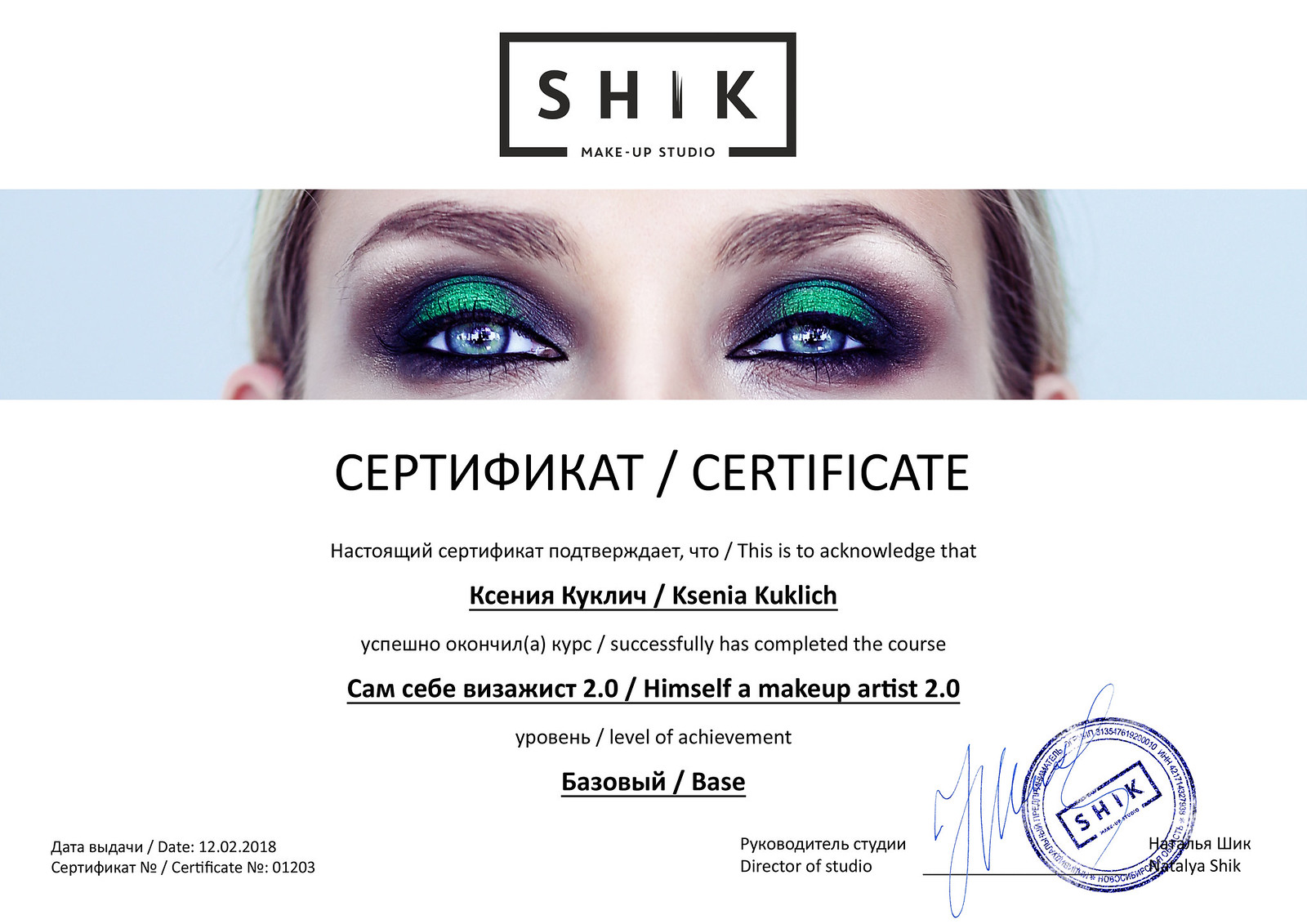This image features a professional makeup artist certificate from SHIK Makeup Studio, prominently displaying its logo in a black square at the top center. Below the logo is an image of a woman's eyes, adorned with metallic green and dark blue smoked-out eyeshadow, highlighting her blue eyes and dark eyebrows, with hints of her blonde and brown hair visible. The certificate is bilingual, likely in Russian and English, and starts with the word "Certificate" in large text. It acknowledges that Ksenia Kuklich has successfully completed the "Makeup Artist 2.0" course at a base level of achievement. At the bottom right, there is a blue circular seal bearing the SHIK emblem, alongside a blue signature from the Director of Studio, Natalia SHIK. The certificate is dated 12-02-2018 and is marked with the certificate number 01203.